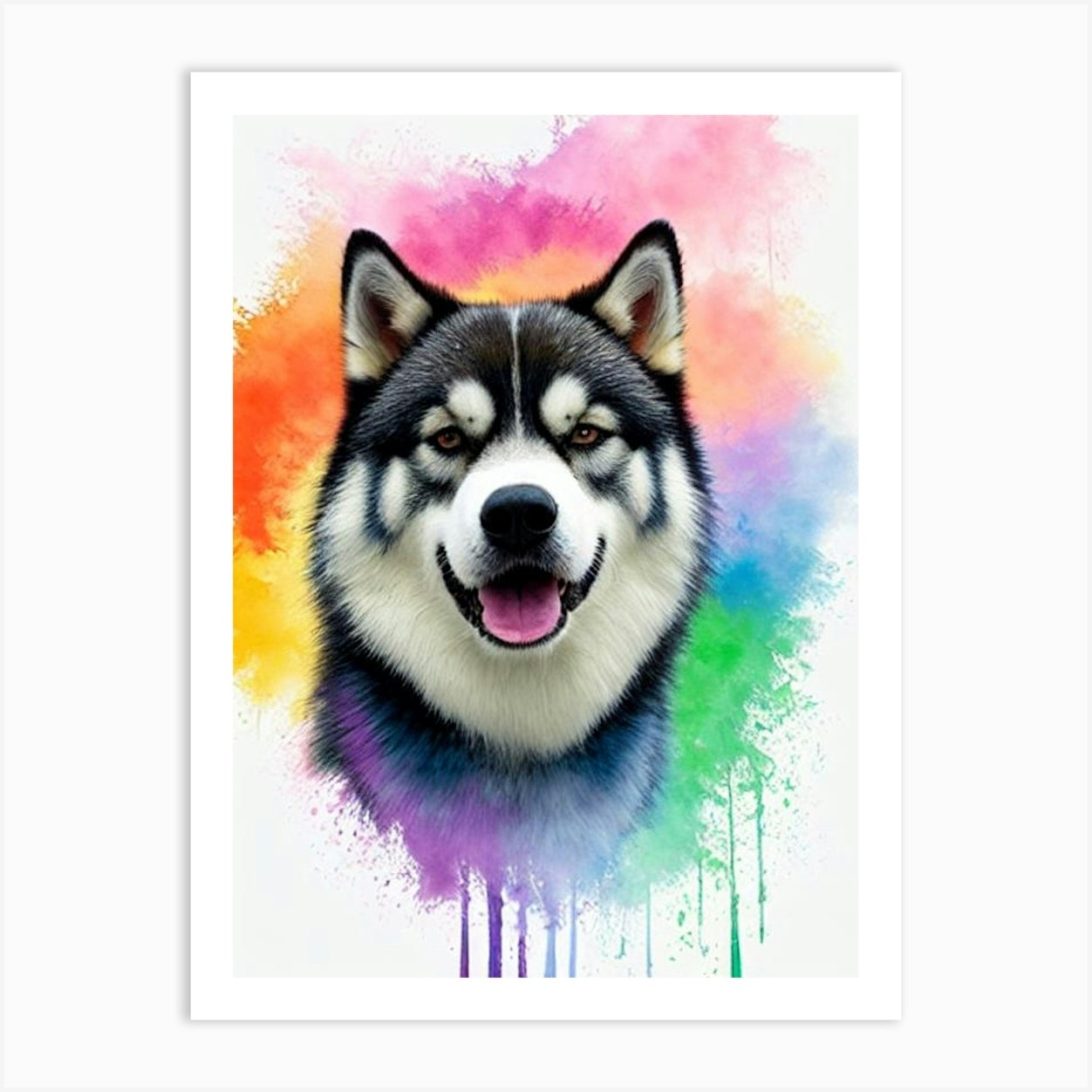The painting, mounted on a white wall with a white frame, features a striking depiction of a Siberian Husky's face in the center. The husky has a distinctive black and white coloration: its chin, nose, and areas around the eyes and inside the ears are white, while the top of its head, part of its neck, and ear tips are black. A unique white line runs down the middle of its head, adding to its Siberian Husky characteristic. The dog’s eyes are a captivating mix of brown or yellow, and its pink tongue is visible, sticking out of its mouth.

Surrounding the husky's head is a vibrant array of colors. Above the dog are splashes of pink, transitioning to orange and reddish hues on the left, then yellow and blue on the right. Below the neck, the painting transitions into a blend of half-purple and half-blue, with some colors dripping down the canvas. Green paint also appears to be dripping down from the right side. The background behind these colors is a light gray, accentuating the lively, watercolor-like paint splatters. The overall effect is a dynamic and colorful portrayal of the husky, framed perfectly within its white border.